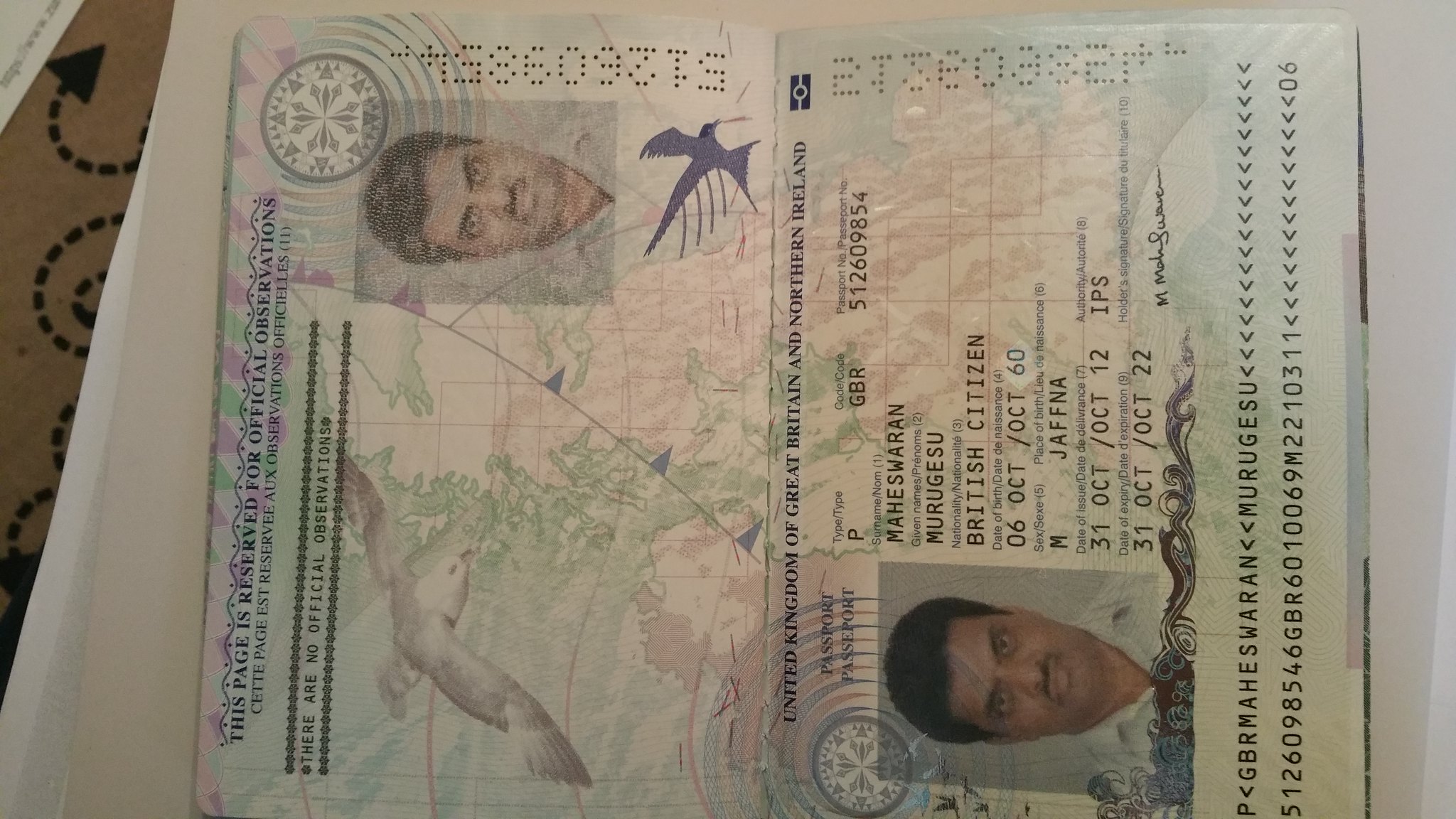The image depicts a sideways view of a British passport belonging to Maheswaran Murugusu. The passport features a formal photograph of Maheswaran, a man with darker skin, short black hair, and a short black mustache. The top of the document prominently reads "United Kingdom of Great Britain and Northern Ireland" in blue text. The passport number is 512609854, and it specifies its type as P, with a color group of GBR.

Maheswaran's personal information reveals that he is a male born on 6 October 1960 in Jaffna. The document includes dates and numbers that are partially obscured but list significant events: 31 October 2012, at 5 p.m., and 31 October 2022. The background of the passport page is adorned with faded images, potentially a map and designs of Europe with birds in flight, along with latitude and longitude lines. The section labelled "This page is reserved for official observation" contains no such observations. The overall appearance of the passport suggests some age due to faded text and images.